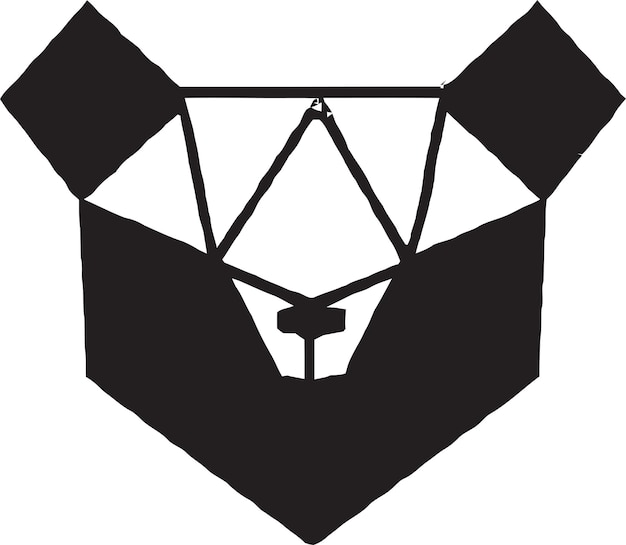The image depicts an abstract artwork against a white background, primarily using black and white colors. The main figure is a large, pentagon-shaped structure with an open top, reminiscent of a box. The pentagon has its pointed V-shape facing towards the viewer, with two lines angling back towards the upper center, forming a symmetrical shape. On the top left and right sides of the image, there are two black squares positioned on their corners at a 45-degree angle, creating a diamond-like appearance. Between these squares are four black shapes resembling a combination of V-shapes or W-shapes. In the center of the pentagon, there's a black pole with a small rectangular box crosspiece. Below this central structure lies an expansive black area. The entire composition has a symmetrical, mirrored quality, with horizontal and angular elements contributing to the geometric abstract design, giving the impression of a digital artwork created with simple drawing tools.